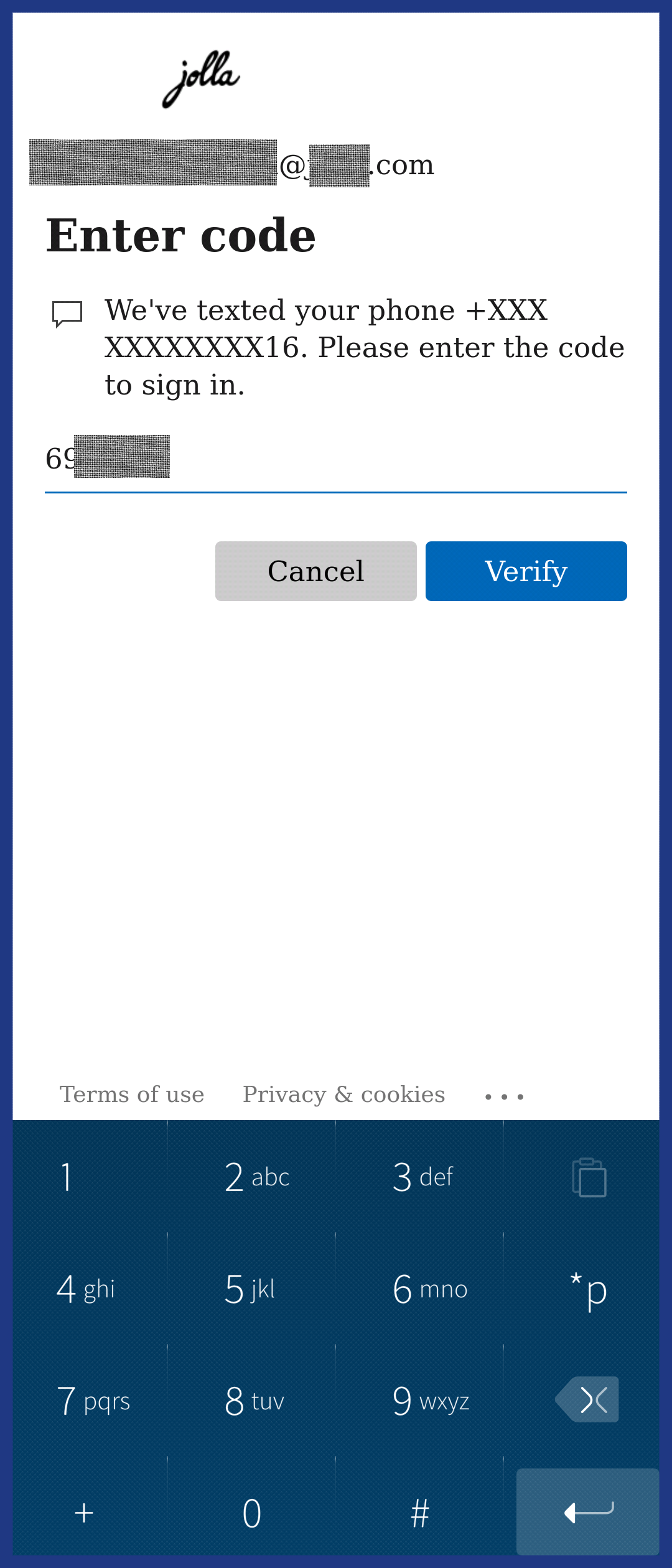The image captures a screenshot from a mobile device, prominently featuring an email login interface from "Jolla." In this screen, the email address is partially redacted, showcasing only the "@" symbol and ".com" with the rest of the address concealed. The message on the screen instructs the user to "Enter the code we've texted your phone" alongside a partially obscured phone number displayed as "+XXXXXXXXXXXXX16." 

The user appears to have begun entering the verification code, with the visible digits "69" followed by a series of blacked-out characters. The redactive elements use a distinct linen-like black and white texture to censor sensitive information.

At the bottom of the screen, two buttons are visible: "Cancel" and "Verify," followed by links to "Terms of Use," "Privacy," and "Cookies." Additionally, there is a horizontal line of three dots indicating more options.

Below these elements, a blue keypad with a traditional phone layout is displayed, featuring white text on a gradient blue background. The keys vary slightly in shades of blue, with some buttons appearing lighter than others.